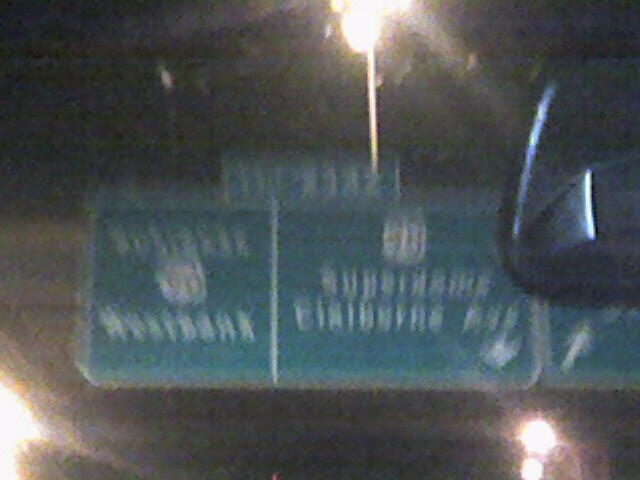This extremely blurry photograph, taken at night from inside a moving car, captures the perspective of either the driver or a passenger through the windshield. Dominating the image is a large green road sign suspended from an overhead bridge, illuminated by a street lamp that casts a bright circle of light above it. The white text and highway symbols on the sign are indistinct due to the blur. In the upper right section of the photo, part of the rearview mirror attachment is visible. Additional streetlights dot the distance, contributing to the scattered lighting in the scene. Framed against the darkness, the overpass looms ahead, enhancing the sense of motion and the nocturnal setting of the highway environment.